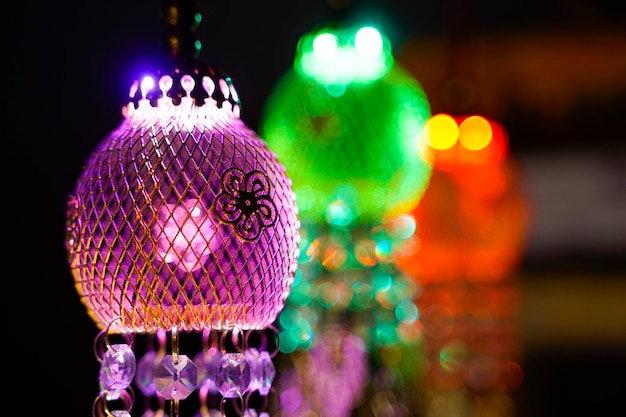The image features a captivating macro photograph of three brightly colored, vintage-style glass lamps set against a black background. The central focus of the photo is a textured glass lamp emitting a vivid purple light, adorned with a decorative flower on its surface and featuring a flower-shaped bulb at its core. This lamp also has metal attachments connecting it to the ceiling and is embellished with hanging glass or crystal elements. To the left of the frame, the prominently displayed purple lamp gives off a slight pink hue, creating a psychedelic feel. Positioned slightly behind and to the right of the purple lamp is a similarly designed green lamp, which appears more blurred but interestingly reflects a purple tint below it. The furthest lamp in the background is red, displaying a neon-like orange and yellow reflection, and is even more out of focus, contributing to a sense of depth. The offset arrangement and increasing blur of the lamps as they recede into the background draw the viewer's eye across the image, creating a modern-yet-nostalgic aesthetic reminiscent of the 70s or 80s.